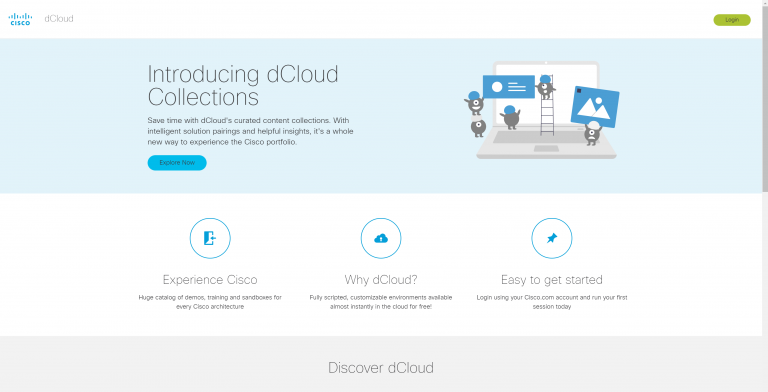The image appears to be a screenshot of a website interface, specifically a section promoting Cisco's DCloud platform. In the top left corner, the Cisco logo is displayed in blue, accompanied by the text "DCloud" in gray. To the top right, there is a green button with black text that reads "Login."

Below the header, there is a light blue banner featuring a prominent gray heading that states: "Introducing DCloud Collections." The banner's body text reads: "Save time with DCloud's curated content collections with intelligent solution pairings and helpful insights. It's a whole new way to experience the Cisco portfolio." Beneath the text, a blue button with black text invites users to "Explore Now."

On the right side of this banner, there is a vector graphic showcasing small, gray, one-eyed creatures holding elements of a web page, seemingly constructing it.

Underneath the main banner, three circular icons are presented:
1. The first circle contains a door icon with the label "Experience Cisco" underneath. The accompanying text elaborates: "A huge catalog of demos, training, and sandboxes for every Cisco architecture."
2. The second circle features a cloud with an upload icon labeled "Why DCloud." The description states: "Fully scripted, customizable environments available almost instantly in the cloud for free."
3. The third circle displays a pin icon with the text "Easy to Get Started." The related text advises: "Log in using your Cisco.com account and run your first session today."

At the bottom of the image, a gray banner urges users to "Discover DCloud."